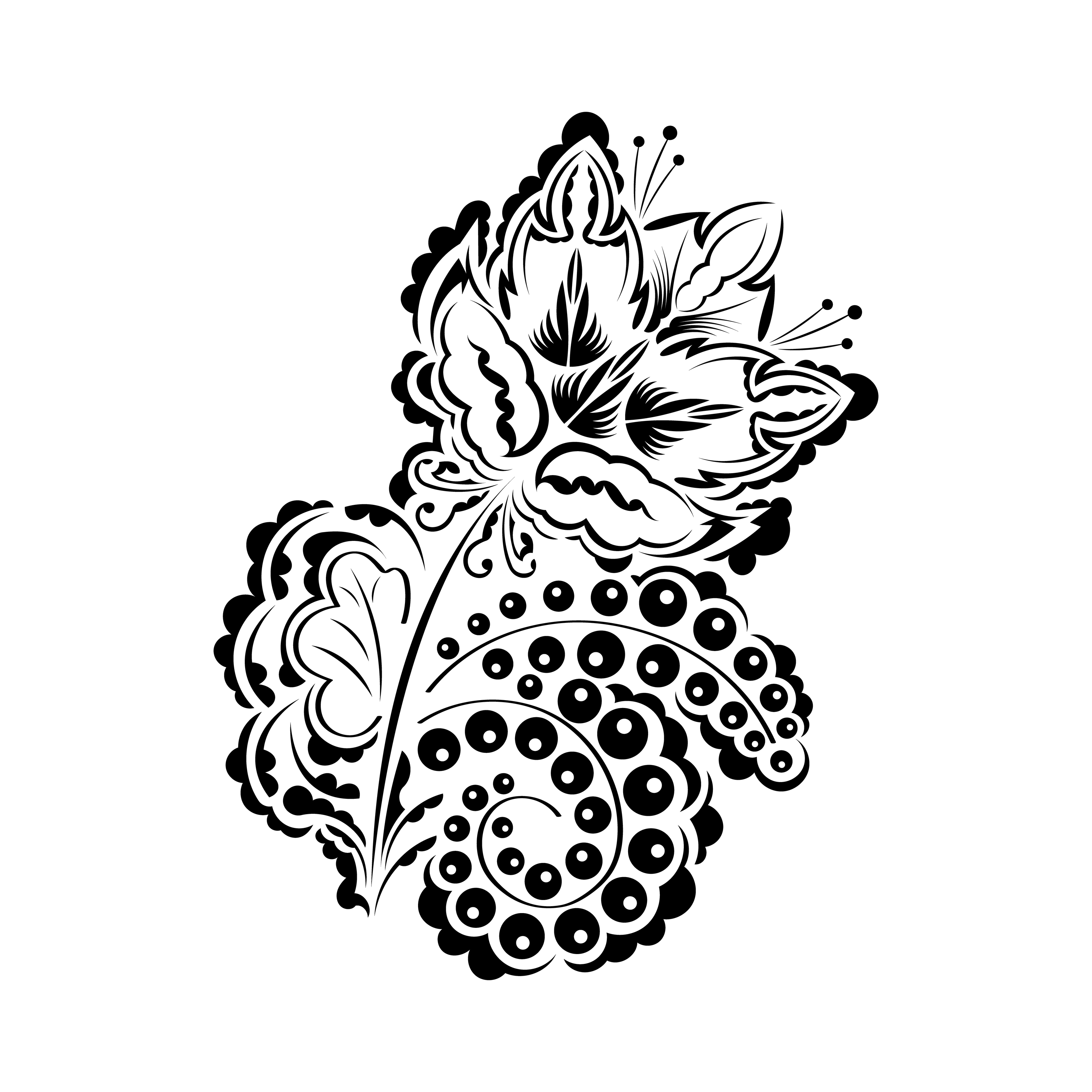This black-and-white clipart image presents a whimsical and abstract floral design, rendered in a cartoony style that resembles a tattoo sketch. At its core, the image features an ornate, irregularly shaped petal cluster emerging from a thin, curving stem. The petals, intricately detailed with scroll-like flourishes and clusters of dots, give the image a dynamic and textured appearance. Extending from the stem are various curlicue shapes and a distinctly patterned leaf with an almost floral texture. One side of the leaf morphs into tentacle-like shapes that spiral and wrap around, adding a sense of surrealism to the piece. The overall composition is symmetrical yet chaotic, with the intricate details creating an illusion that, when observed closely, hints at various forms—such as octopus tentacles or even the silhouette of a cat’s head with ears perked up. This abstract representation blends elements of nature with imaginative twists, culminating in a captivating and multifaceted floral design.